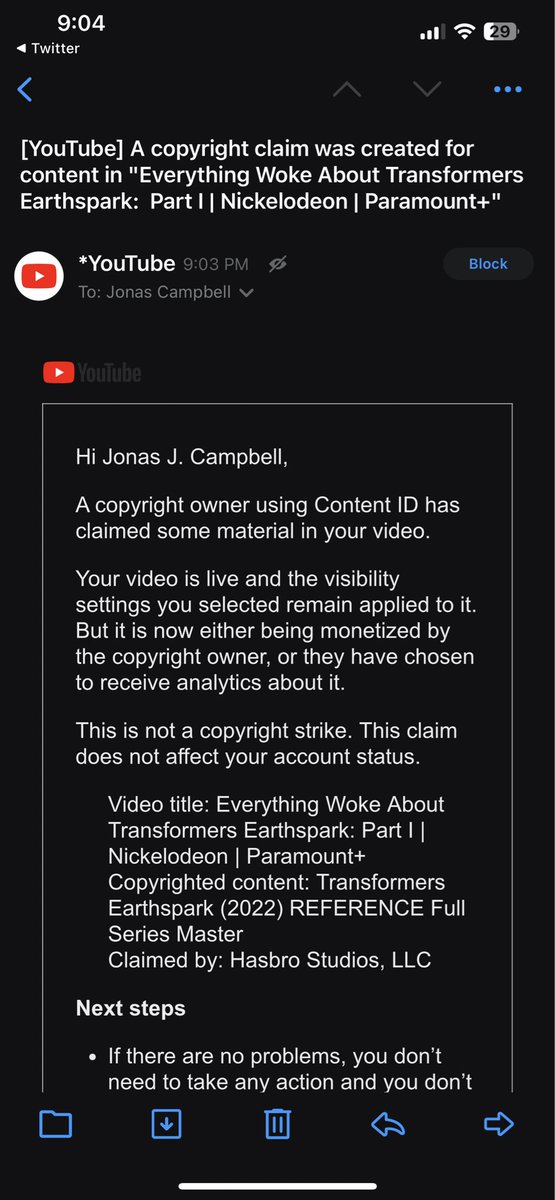**Detailed Caption:**

The image depicts a cell phone screen, which is a tall rectangle with a black background. At the top-left corner, the time "9:04" is displayed in white. On the top-right corner, there are three white icons: a three-bar signal strength indicator, a three-indicator Wi-Fi signal, and a horizontal battery icon showing a 29% charge. 

Just below the time, on the left side, you see "Twitter" along with a left-facing caret in small letters. Below it, there's a prominent left-facing caret in blue. Moving to the right side, a grayed-out upward caret and a grayed-out downward caret are visible, followed by three horizontal blue dots on the far right. 

The central part of the screen displays what appears to be an email from YouTube regarding a copyright claim. The email subject reads, "[YouTube] A copyright claim was created for content in 'Everything Woke About Transformers Earthspark: Part One | Nickelodeon | Paramount Plus'." Below this, the YouTube play icon is represented by a white circle enclosing a red square with a right-facing white caret.

The sender is identified in white text as "*YouTube," and the timestamp "9:03 PM" is shown in gray to the right. Further right, there's a blue "Block" option. 

Following this, in gray text, it states, "To Jonas Campbell" accompanied by a downward arrow. Directly beneath, the red YouTube logo is displayed next to the word "YouTube" in gray, all enclosed within a gray-outlined vertical rectangle containing the email content.

The email body, in white text, begins: "Hi, Jonas J. Campbell. A copyright owner using Content ID has claimed some material in your video. Your video is live, and the visibility settings you selected remain applied to it, but it is now either being monetized by the copyright owner, or they have chosen to receive analytics about it. This is not a copyright strike. This claim does not affect your account status." An indented section then follows: "Video title: Everything Woke About Transformers Earthspark, Part One, Nickelodeon, Paramount Plus. Copyright content: Transformers Earthspark (2022). Reference: Full Series Master. Claimed by: Hasbro Studios, LLC."

The email continues with "Next steps" in bold white text and offers a bullet point that says, "If there are no problems, you don't need to take any action," but the remaining text is cut off.

At the very bottom of the screen, a blue icon panel shows symbols for a file folder, a downward arrow (indicating download), a trash can, a left arrow, and a right arrow.